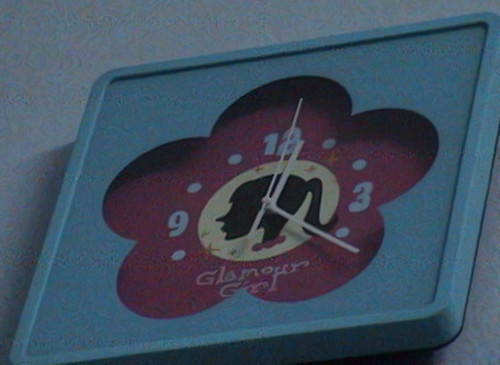This color photograph showcases a close-up view of a square wall clock mounted on a slate grayish-blue wall. The clock is turquoise blue, both in its outer frame and its interior background. At the center of the clock's face, a striking outline of a five-petal flower in light red is prominently displayed, with a vivid yellow circle marking its center. Superimposed on this design is the silhouette of a woman with a ponytail, along with the inscription "Glamour Girl" underneath. The clock features only the numbers 12, 3, and 9, while the other hours are indicated by dots. The time is displayed with yellow hour, minute, and second hands, pointing to approximately 12:21.